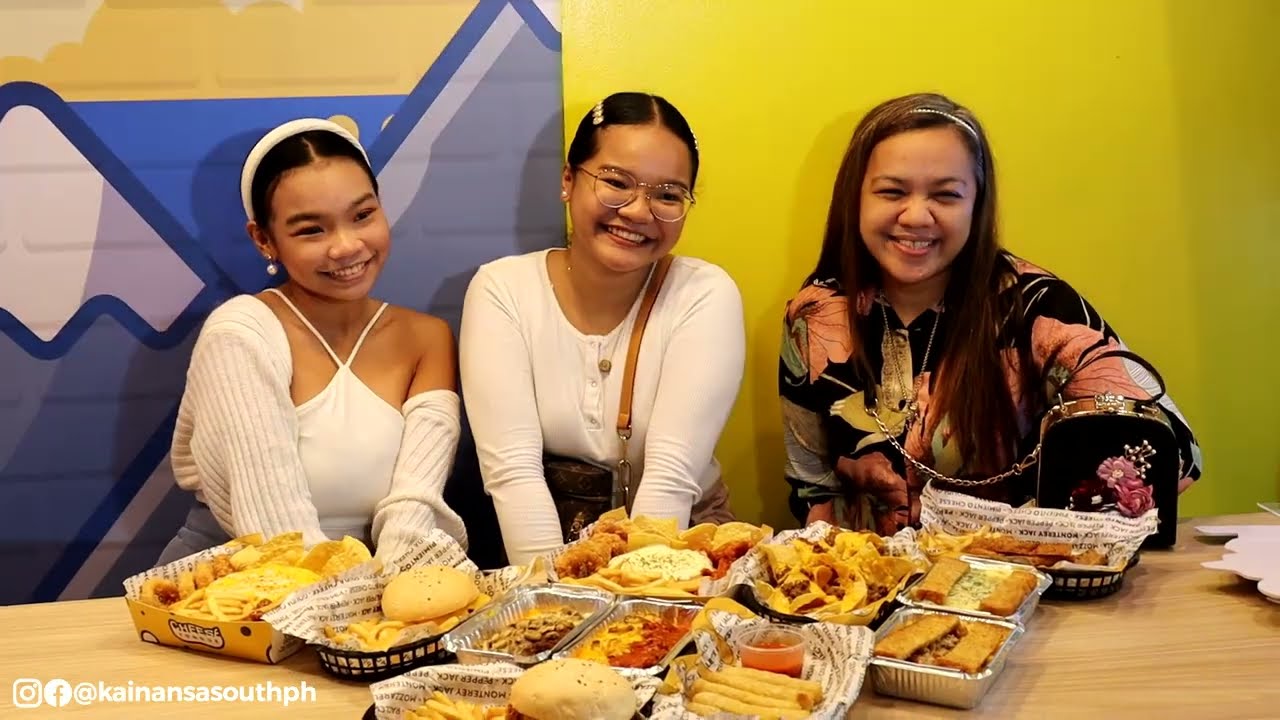Three women, all of apparent Asian descent, are seated at a wooden table loaded with an abundant spread of food, including foil trays and baskets containing burgers, nachos, cheese sticks, french fries, and more assorted items. The woman on the left, younger in appearance, is wearing a white top with a white headband and small dangle earrings, her dark hair pulled back and smiling at the camera. The middle woman, also smiling and wearing glasses, is dressed in a white long-sleeved shirt with a brown strap over her left shoulder indicative of a purse. The woman on the right, seemingly older, wears a colorful floral-patterned blouse and a thin silver headband, her long brown hair cascading over her shoulder. A small floral-adorned black purse sits on the table in front of her. Behind them, the wall backdrop is split into two, with the right side painted solid yellow and the left side featuring a mural of cartoony snow-capped mountains against a blue sky.